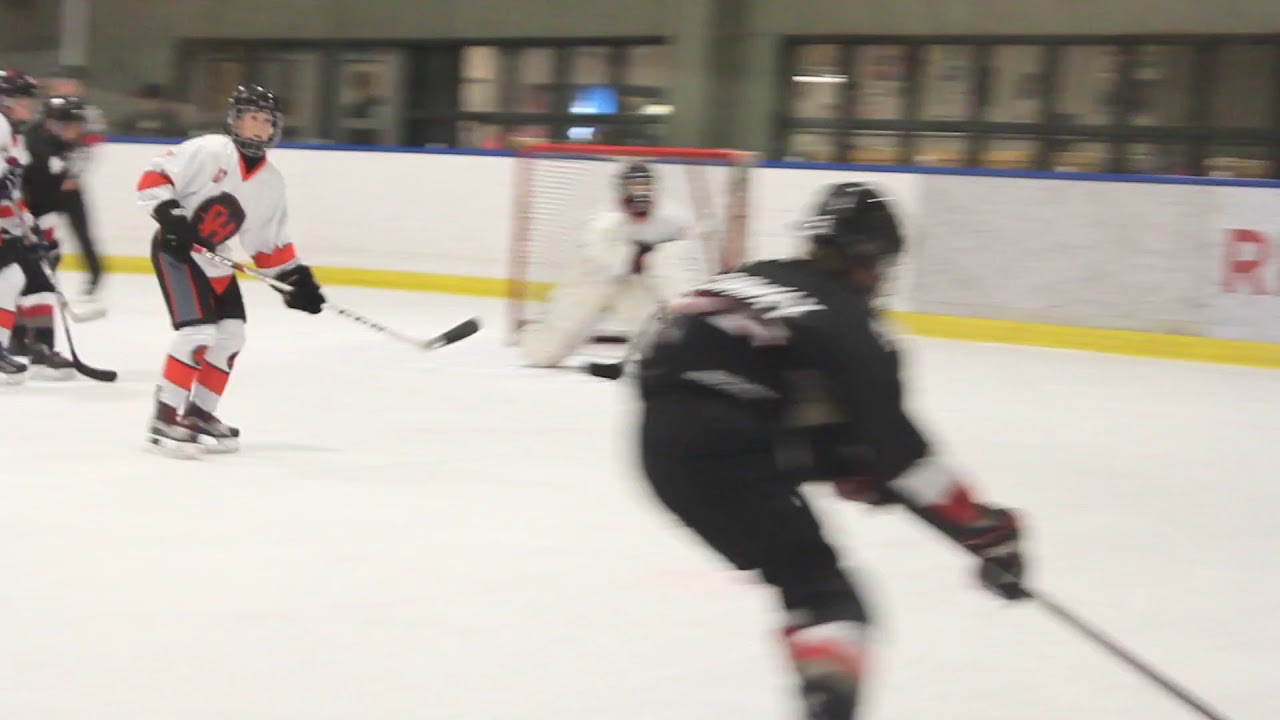The image captures an intense moment in a hockey game at a rink, featuring two teams distinguishable by their uniforms: one predominantly in black, and the other in white and red. The focal point is a player in a black uniform, positioned at the bottom right, speeding towards the goal with his hockey stick extended, ready to take a shot. There's noticeable motion blur around him, indicating his swift movement. Two defenders from the white and red team, along with their goaltender, are in the top left, bracing for the incoming attack. The goaltender is visibly prepared to parry the shot. In the background, behind the hockey net, there's a barrier and a set of see-through windows, adding depth to the scene. Another player from the black team is visible on the left, seemingly moving in to assist with the offensive play.